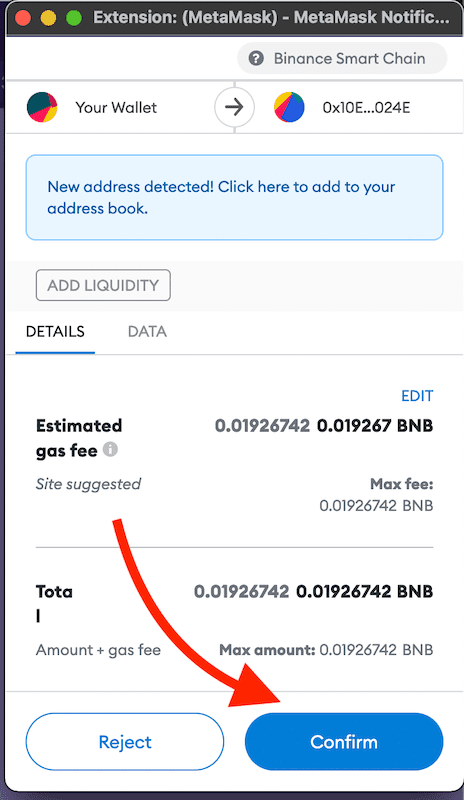Screenshot of a cryptocurrency wallet interface, likely within a Binance Smart Chain application running on a Mac operating system. The top of the interface features the Mac OS window controls: a red circle, yellow circle, and green circle on a grey bar. The title bar reads "Extension (MetaTask) - MetaTask Notification" in white text.

Below the title bar is a menu that includes a grey circle with a white question mark, labeled "Binance Smart Chain" in grey text. Adjacent to this menu is a multicolored circle composed of yellow, pink, blue, and red segments, followed by an address abbreviation "0x10E...024E."

A light blue text box below these elements states, "New address detected. Click here to add your address book." Further down, there's a light grey tab labeled "Add Liquidity." Next to it, the "Details" tab is selected, with additional tabs for "Data" and "Estimated Gas Fee" available for selection.

A prominent red arrow points from the section to the "Confirm" button, with an option to "Reject" next to it. The bottom section displays various amounts for transaction fees, including a maximum fee and the total amount plus gas fee.

This detailed description captures the interface elements and their layout, providing a comprehensive understanding of the wallet's screenshot.